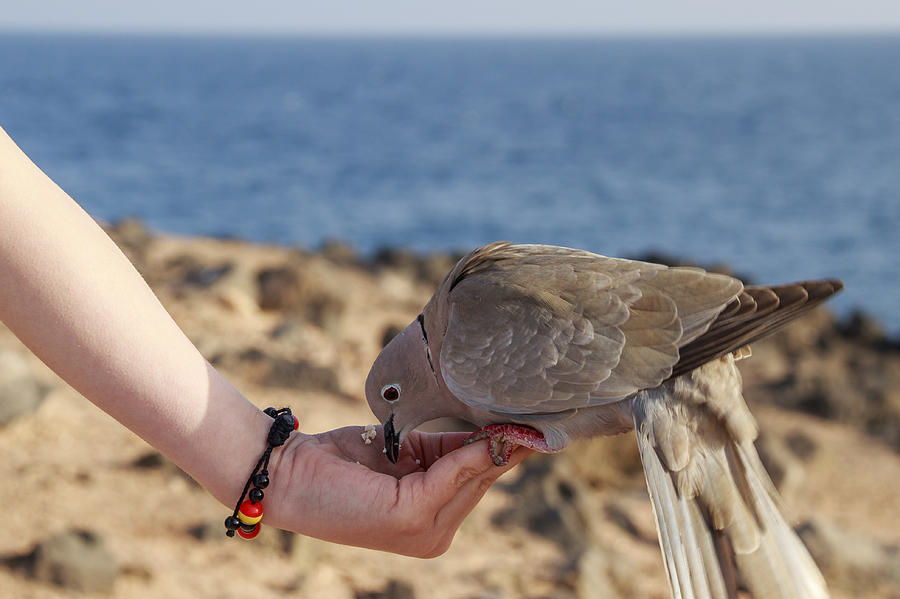This detailed photograph captures a serene moment of a light beige dove-like bird feeding from the outstretched hand of a young Caucasian woman. The bird, with a distinct mix of tan and white tail feathers, delicately pecks at what appears to be popcorn or a white grain. The woman, identified by her pale skin and a beaded bracelet featuring a black cord with orange, yellow, and black beads, extends her hand from the upper left corner in a scooping motion. Behind this tender interaction, the distant, out-of-focus coastline reveals a scenic backdrop of blue ocean waters, light brown sand, and dark green bushes, providing a tranquil beach setting.